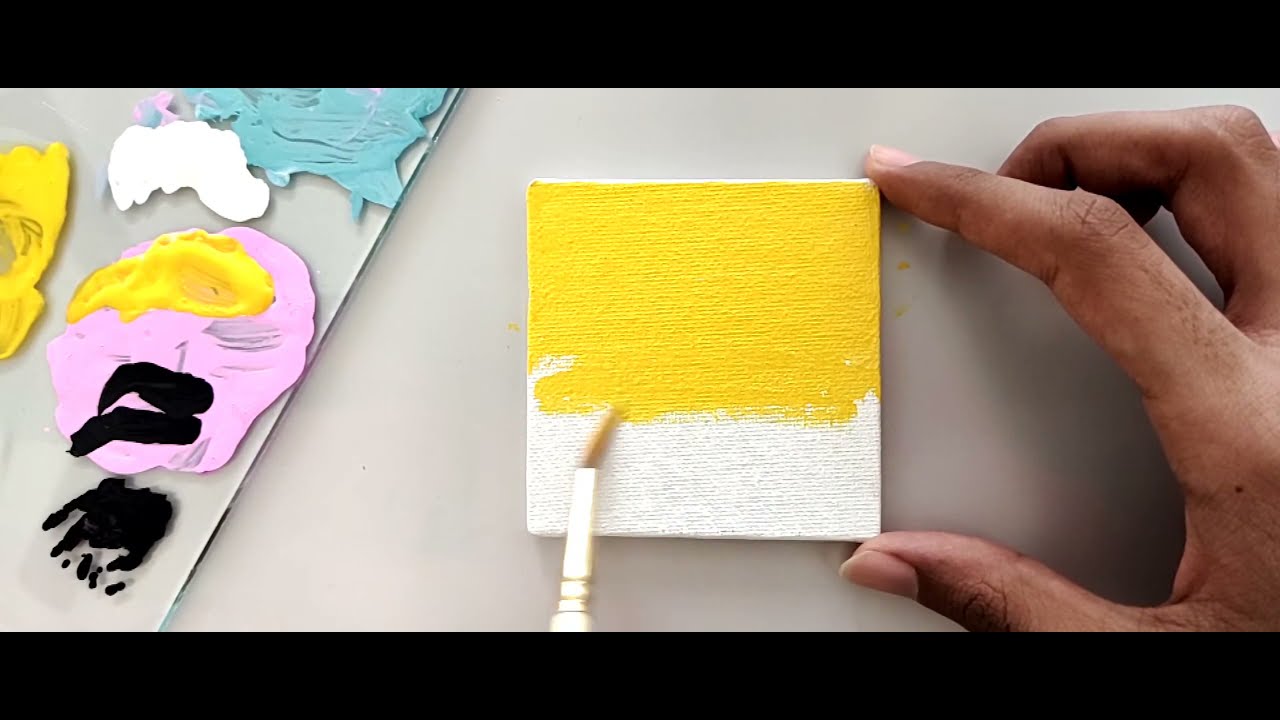In a horizontal, rectangular image, we see a white square canvas held by a person with a dark-skinned right hand, their thumb and index finger gripping the top and bottom edges of the canvas. Half of the canvas is already painted in vibrant yellow paint, with the remaining half still white. A paintbrush, coming from the bottom of the image, is actively adding more yellow paint onto the canvas. The background features a gray surface, likely a table or desk. To the left of the canvas, there is a flat palette with an array of pastel paints: light blue, light purple, yellow, black, and white, all squeezed out in small amounts on the gray surface. The image is bordered by horizontal black stripes at the top and bottom, each about an inch wide.